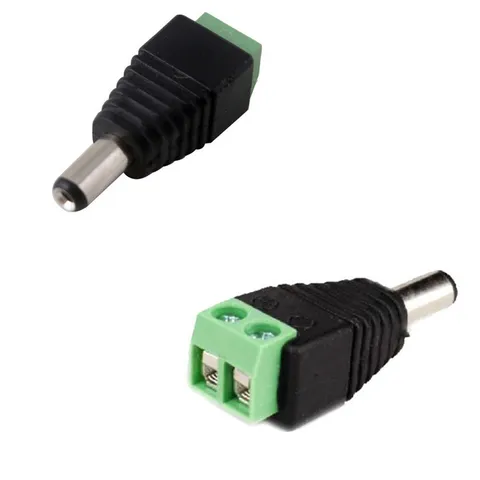The image features two electronic components set against a plain white background, presented from different angles. The components consist of a black cylindrical cover that tapers into a silver tube-like end, resembling the connector of a power cable. The wider end of the black cylinder has a distinct light green plastic piece with metal holes, presumably for plugging in wires or connecting to another device. Together, these elements suggest that the objects are part of an electronic connector or adapter, hinting at a versatile and adjustable nature for connecting various electronic cables or plugs.